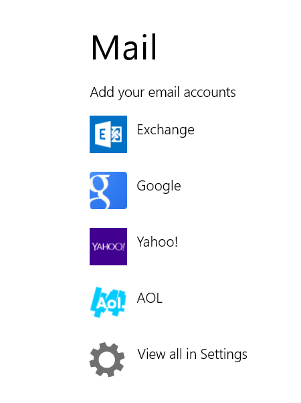This horizontal screenshot displays a "Mail" category on a smartphone. A thin light gray line runs across the top of the image, while the background remains white with no additional border. At the top, the word "Mail" appears in large, bold black font. Below, smaller black text instructs users to "Add your email accounts."

The image features a vertical list of five icons, each corresponding to different email providers:

1. **Exchange**: Represented by a blue and white square icon with the letter "E."
2. **Google**: Marked by a blue square containing a lowercase "g" in white.
3. **Yahoo**: Indicated by a purple square with the capitalized text "YAHOO" in white.
4. **AOL**: Displayed with a logo consisting of white text on a light blue squiggle, not enclosed in a square.
5. **View in All Settings**: Accompanied by the familiar gray gear icon.

This detailed depiction highlights the interface's clean design and intuitive layout, aiding users in managing their email accounts efficiently.